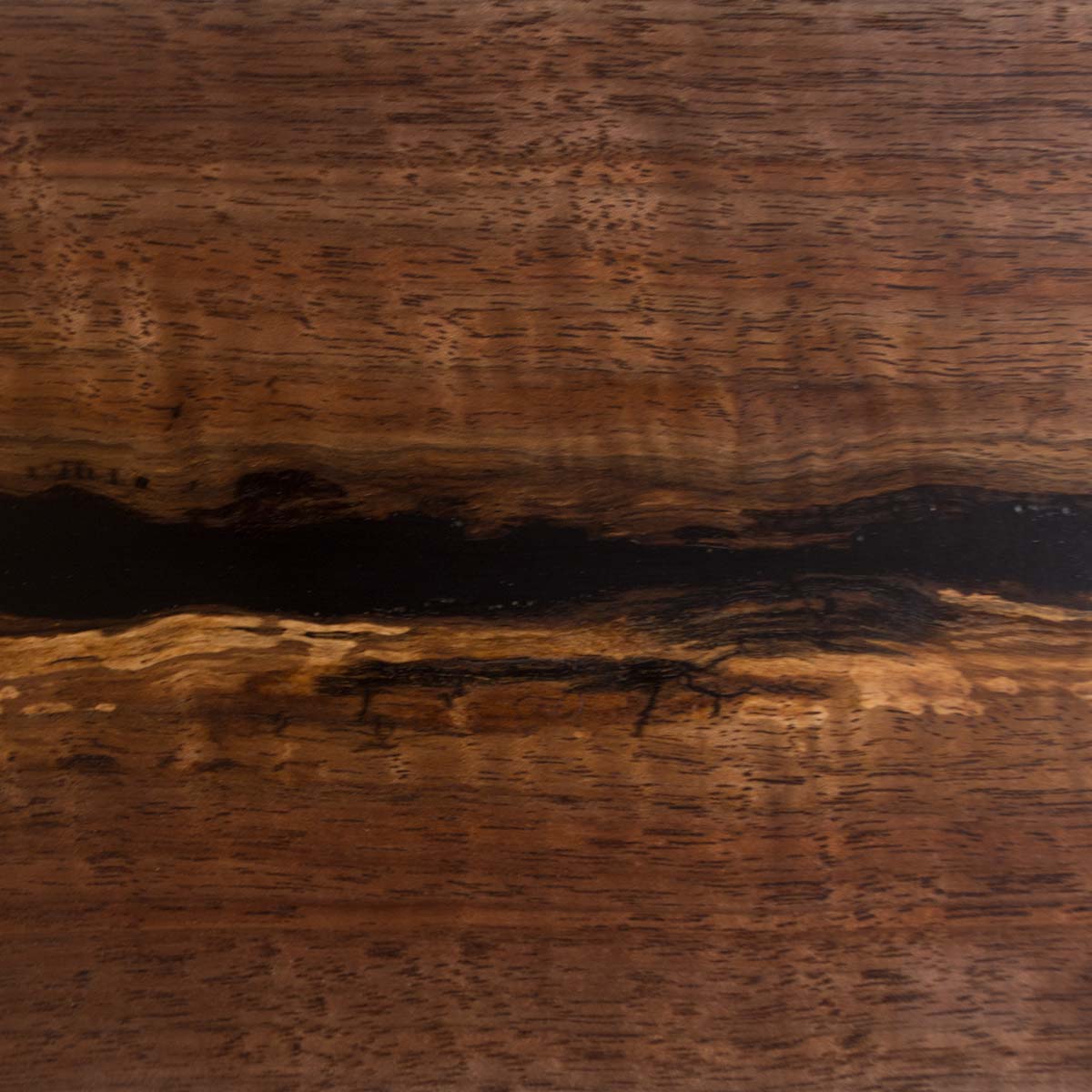This close-up image captures the intricate details of a piece of wood, presenting a fascinating interplay of colors and textures. At the center, a prominent, dark, wavy line—likely a crack or an area of wood rot—extends horizontally, effectively dividing the wood into two distinct sections. This dark band is accompanied by tiny, wave-like black grains that accentuate the natural patterns of the wood. The wood itself displays a rich spectrum of colors, ranging from light beige to deeper orange-brown hues, interspersed with darker brown lines that highlight its layered structure. Despite the image being somewhat blurry, the rough texture and natural, possibly cut-out formation of the wood are clearly evident, showcasing the beauty and complexity of its grain.